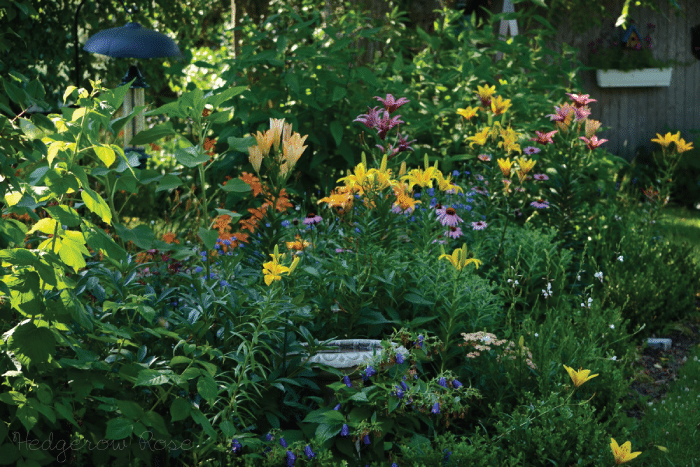This photograph depicts a beautifully overgrown backyard garden, reminiscent of a wild, cultivated sanctuary of native plants. The scene bursts with a myriad of wildflowers in myriad hues: brilliant yellows, delicate pinks, fiery oranges, striking purples, and soft blues. Amongst the dense foliage and tall flowers—some reaching four to five feet in height—stand recognizable species such as hollyhocks, daisies, cone flowers, and tiger lilies. At the garden's heart lies a gray, concrete birdbath, partially obscured by the towering flora. In the background, you can discern a house, its wooden paneling, or perhaps barn-like structure, painted in black clapboard with hints of white, and adorned with a long basket of flowers hanging on its side. Adding to the rustic charm, a tall lamppost with a black covering peaks from the flowered canopy, and a bird feeder is just visible in the top left corner. This vibrant, nature-embraced garden creates a serene, untamed refuge.